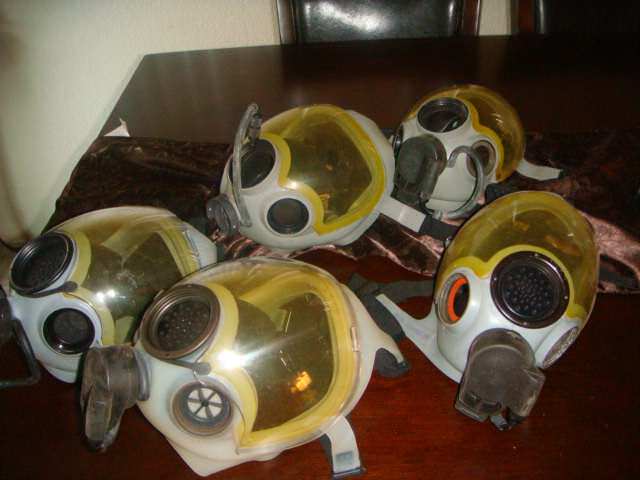This close-up photograph captures five gas masks laid out on a dark brown finished wooden table. Each gas mask features a gray, rubbery bottom portion that houses a black filter canister. The photos also show a respirator section in silver, with the eye shield being a distinctive opaque yellow. The masks seem designed to cover the entire front of the head, and their curved front contours hint at comprehensive face coverage. Black straps are visible, likely used to secure the masks over the head. In the background, two dark brown wooden chairs with black cushions on their backs can be seen, adding context to the scene. The detailed structure and multiple filter attachment points suggest these masks could be for sophisticated tasks such as working in smoky or chemical-heavy environments.